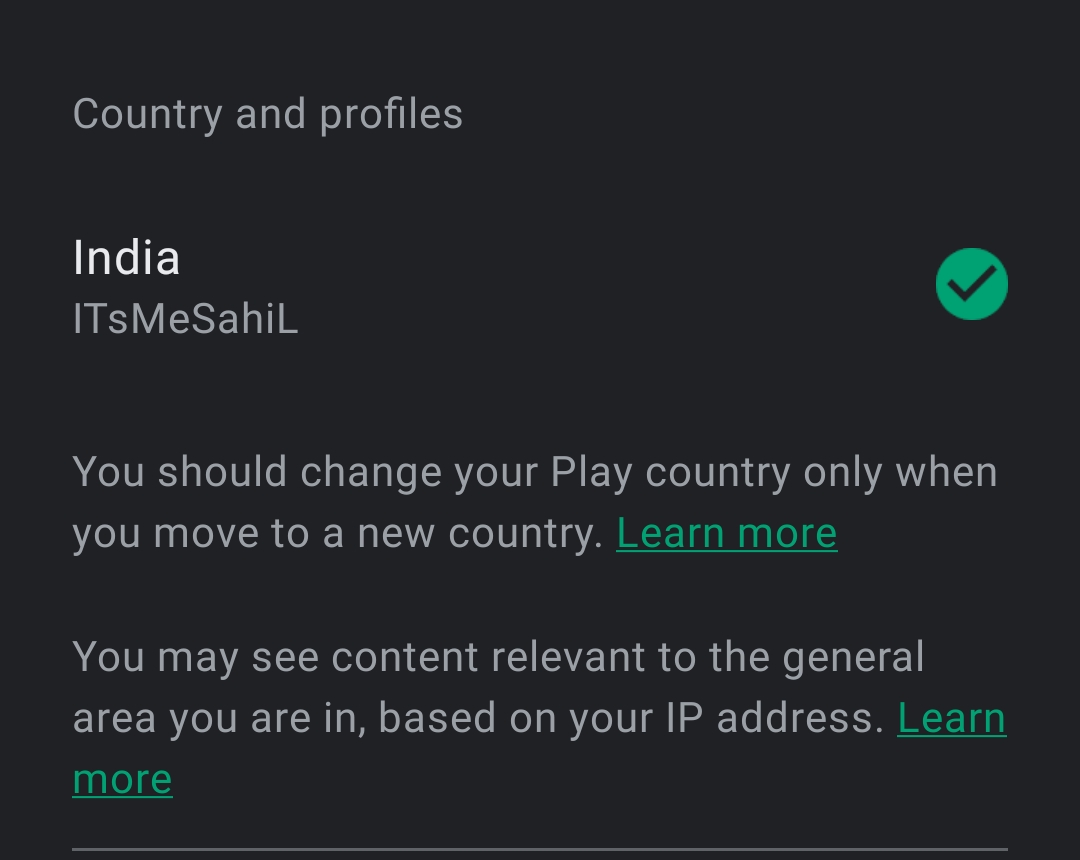This image depicts a screenshot in dark mode, characterized by a charcoal gray background. In the upper left-hand corner, light gray text reads "Country" and "Profiles." Below that, aligned to the left, the word "India" appears in white. On the right side, a green circle with a charcoal gray checkmark inside is visible.

Underneath "India," in smaller gray text, the phrase "IT'S ME S A H I L" is displayed with the capital letters "ITS" and "S A H I L" interspersed with lowercase letters. Following this text, a sentence in gray reads, "You should change your play country only when you move to a new country." To the right, the words "Learn more" appear as a clickable green text link.

Further down, another line in gray states, "You may see content relevant to the general area you are in, based on your IP address." Again, the phrase "Learn more" appears as a green text link.